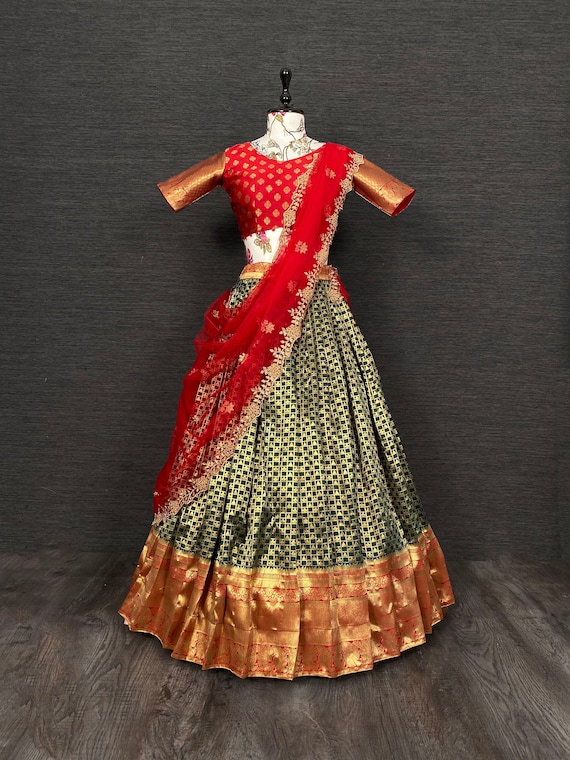This photograph features a detailed, floor-length gown displayed on a mannequin with a white body and a black knob for a head. The backdrop is a textured, dark grey wall, contrasting with the light brown wooden floor beneath. The gown has a vivid red bodice adorned with gold diamond patterns and metallic orange short sleeves that extend outward. Draped from the left shoulder down to the right side is a striking red sash, embellished with white lace along its edges and evenly spaced white symbols. The skirt of the dress transitions into a checkered pattern of light black and white dots, culminating in a thick, gold hem. The mannequin’s color schemes, particularly its arms and neck, complement the gown's elegance and intricate design, suggesting an exhibit-worthy garment that could be displayed in a museum.